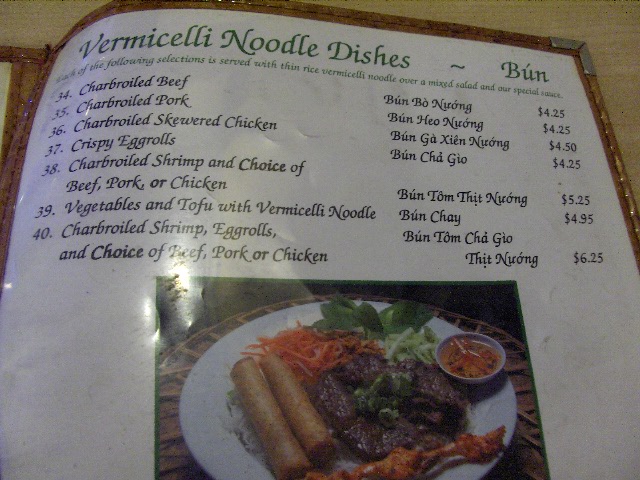In this detailed image, we see the inside of a menu presented against a light brown table. The menu itself features a crisp white background encased within a brown, leather-like plastic cover that is neatly folded, stitched together, and adorned with metal brackets at the corners for added durability. This protective design encloses the menu in clear plastic, giving it a clean and polished appearance.

At the bottom of the image, there is a photograph of one of the menu items, framed by a green border. The dish is attractively presented on a plate that sits atop a rustic platform made of several wooden sticks. The food arrangement includes two spring rolls, a generous serving of shredded carrots, a scattering of fresh spinach leaves, and a portion of dark brown meat garnished with broccoli. Accompanying these items is a small white dish containing an orange substance, and beneath it all, there is a skewer with grilled meat.

The top of the menu prominently displays the title "Vermicelli Noodle Dishes" in green text, followed by a tilde and the Vietnamese term "Bún." Although part of the text is blurred and difficult to read, the menu explains that each dish is served with thin rice vermicelli noodles, a mixed salad, and their special sauce. The dishes are sequentially numbered from 34 to 40, including both the English names and their Vietnamese equivalents, along with the prices:

34. Charbroiled Beef - "Bún Bò Nướng" - $4.25
35. Charbroiled Pork - "Bún Heo Nướng" - $4.25
36. Charbroiled Skewered Chicken - "Bún Gà Xiên Nướng" - $4.50
37. Crispy Egg Rolls - "Bún Chả Giò" - $4.25
38. Charbroiled Shrimp with Choice of Beef, Pork, or Chicken - "Bún Tôm Thịt Nướng" - $5.25
39. Egg Rolls and Tofu with Vermicelli Noodles - "Bún Chả Đậu" - $4.95
40. Charbroiled Shrimp, Egg Rolls with Choice of Beef, Pork, or Chicken - "Bún Tôm Chả Giò Thịt Nướng" - $6.25